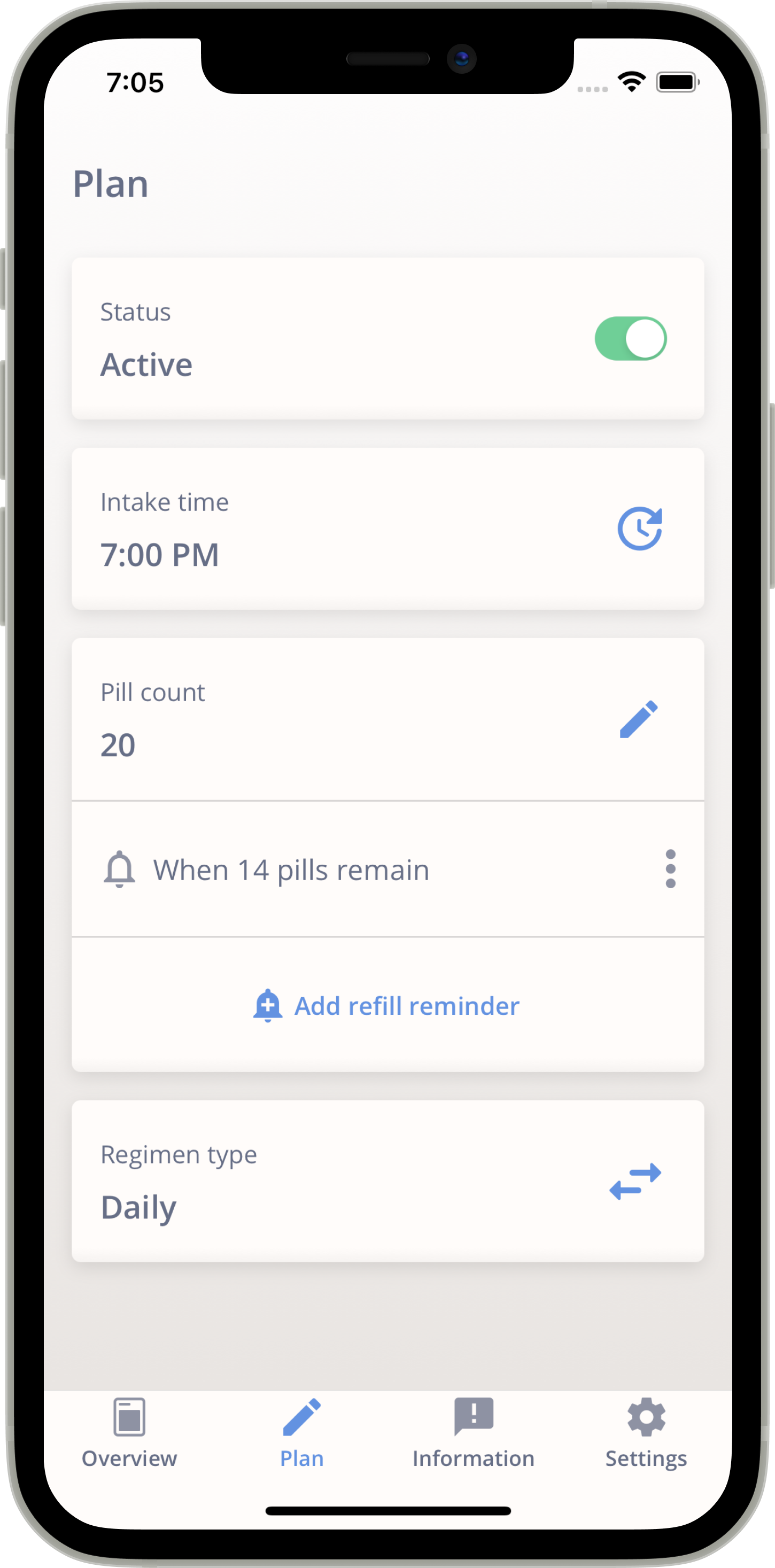A sleek black mobile device, potentially a tablet, is depicted displaying a medication management application. The time "7:05" is prominently displayed in the upper left corner, while Wi-Fi and battery icons are on the upper right. The device’s screen is predominantly white, featuring the word "Plan" at the top. Below this, a series of long, thin rectangles present various information fields. 

The first field indicates "Status: Active," toggled on and highlighted in green. The "Intake Time" is set to "7 p.m." with a blue clock icon situated beside it. The subsequent field lists a "Pill Count: 20," accompanied by a blue pencil icon for editing. Further down, it mentions a notification setting: "When 14 pills remain," marked with a bell icon and a three-dot vertical menu on the side. 

Another entry displays "Add Refill Reminder" next to a bell icon with a plus sign. Under "Regimen Type," it specifies "Daily," with dual arrows pointing right and left highlighted in blue. 

At the very bottom, the screen’s navigation menu shows "Overview," "Plan Information," "Settings," with "Plan" highlighted in blue while the others are in gray. A black line divides this menu from the rest of the screen contents. This interface suggests the device is running a sophisticated medication management application.